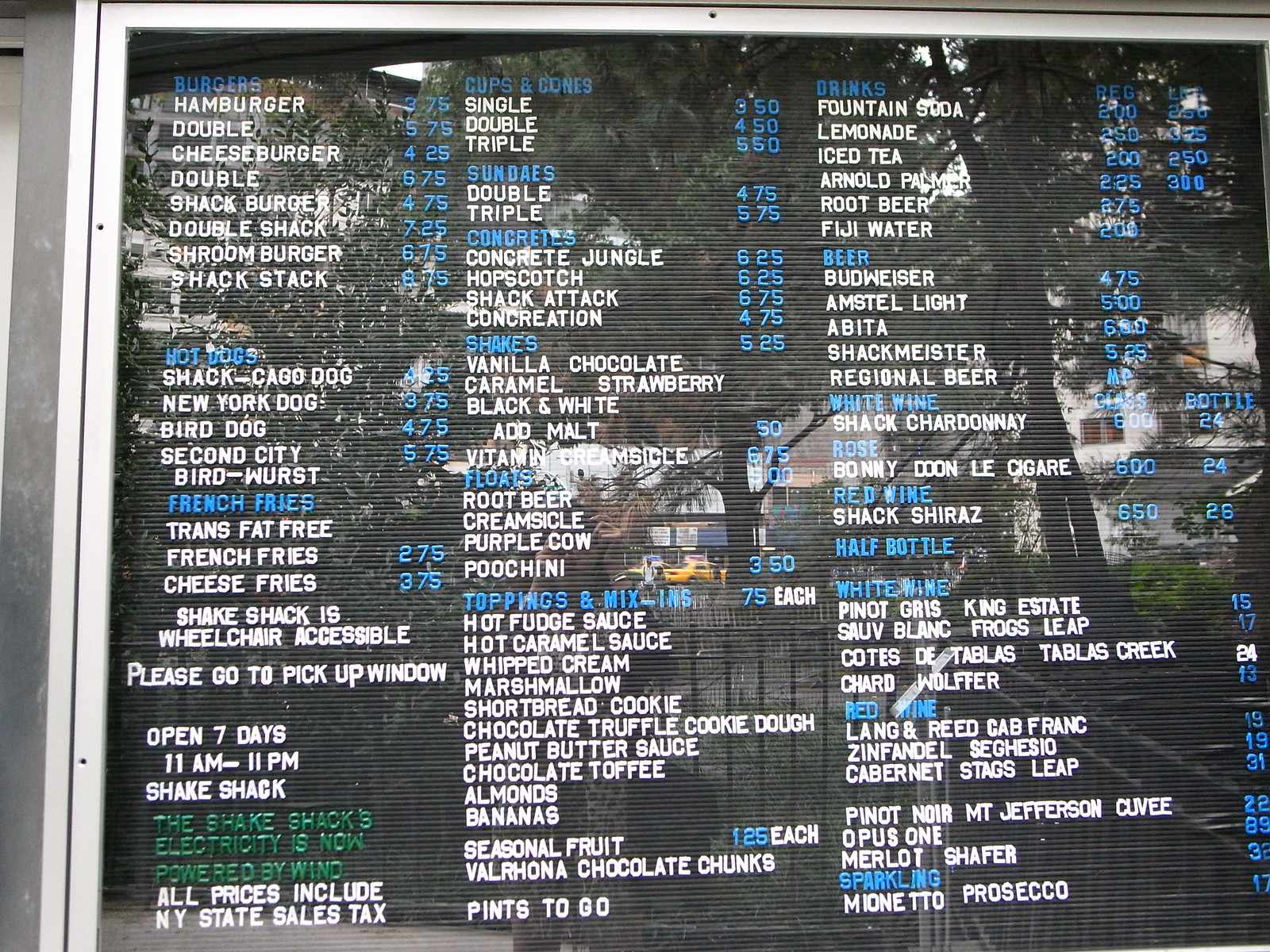This image features a detailed Shake Shack menu board. Prominently displayed at the bottom left corner, the text highlights that Shake Shack's electricity is now generated by wind power, written in green font. The operational hours are noted as being open 7 days a week from 11 a.m. to 11 p.m. The menu board utilizes a system of attachable letters and numbers under a protective glass overlay, allowing for easy updates. The menu categories include burgers, hotdogs, french fries, cups and cones, sundaes, concretes, shakes, floats, toppings, and mix-ins. All prices listed include New York State sales tax.